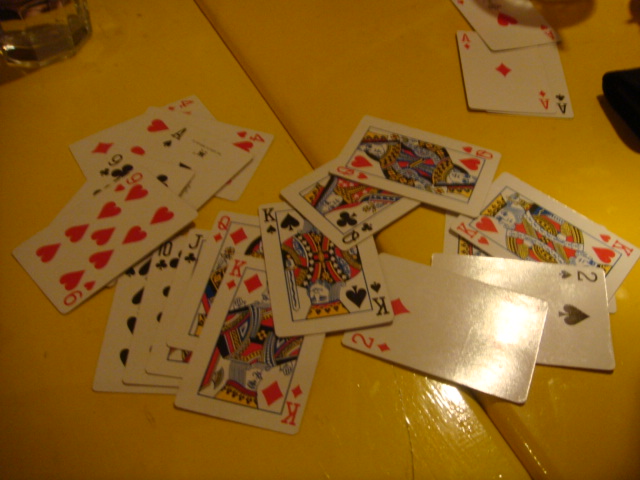In this overhead image, we see an intricate scene on two yellow tables pushed together, creating a vibrant backdrop for a scattered deck of playing cards. At the center, the Queen of Clubs lies horizontally between the table lines, topped at an angle by the Queen of Hearts. Additional cards are visible—faced up—across the scene, with clusters on the left and right sides of the tables. The top left corner of the image captures the base of an octagonal glass with raised edges, adding texture and depth. On the right, the corner of a black cell phone peeks into frame. The left side of the photograph is shrouded in shadow, while the bottom right corner is brightly illuminated, casting a reflective sheen on two prominent cards: the Two of Diamonds and the Two of Clubs. The light's glare bounces off these cards and onto the table to their left, enriching the image with a dynamic play of light and shadow.